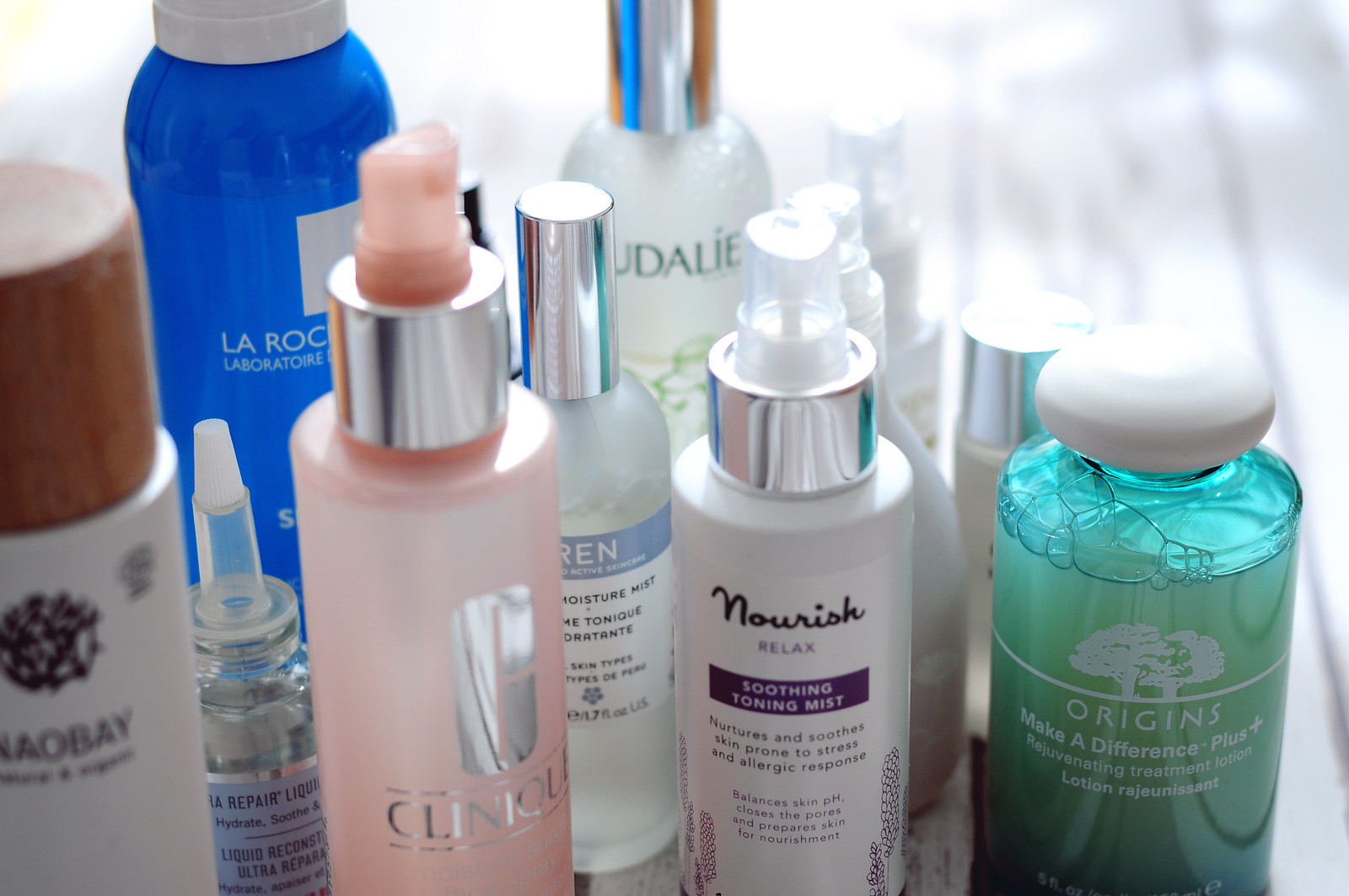The image captures an array of cosmetic bottles prominently arranged against a pale gray and white, slightly blurry background. Dominating the lower right corner is a vibrant green bottle with a flat white screw cap, resembling a stopper, inscribed with a white tree logo and the word "Origins" in white lettering below it. Adjacent to it on the left is a sleek white bottle with a silver and clear spray pump, adorned with purple lettering that reads "Nourish."

Behind these, partially hidden, are shorter bottles featuring white bodies and silver caps. In the lower left corner, a slightly blurry white bottle with a large brown snap-on cap stands out, marked with black or dark purple writing.

Near the upper left corner, a royal blue bottle glistens with reflections of its neighboring bottles. Its partially visible white cap at the top edge of the image bears white lettering spelling "La Roche Laboratory" within a white square, though only "L-A-R-O-C" is visible.

In the foreground, to the right of the brown-capped bottle, is an elegant pink glass bottle with the "Clinique" logo in silver lettering, topped with a silver cap and a plastic spray pump. Centrally positioned are two additional bottles, either white or clear, each capped with silver tops. The detailed arrangement of these bottles, capturing both brand and style, presents a comprehensive showcase of cosmetic products.